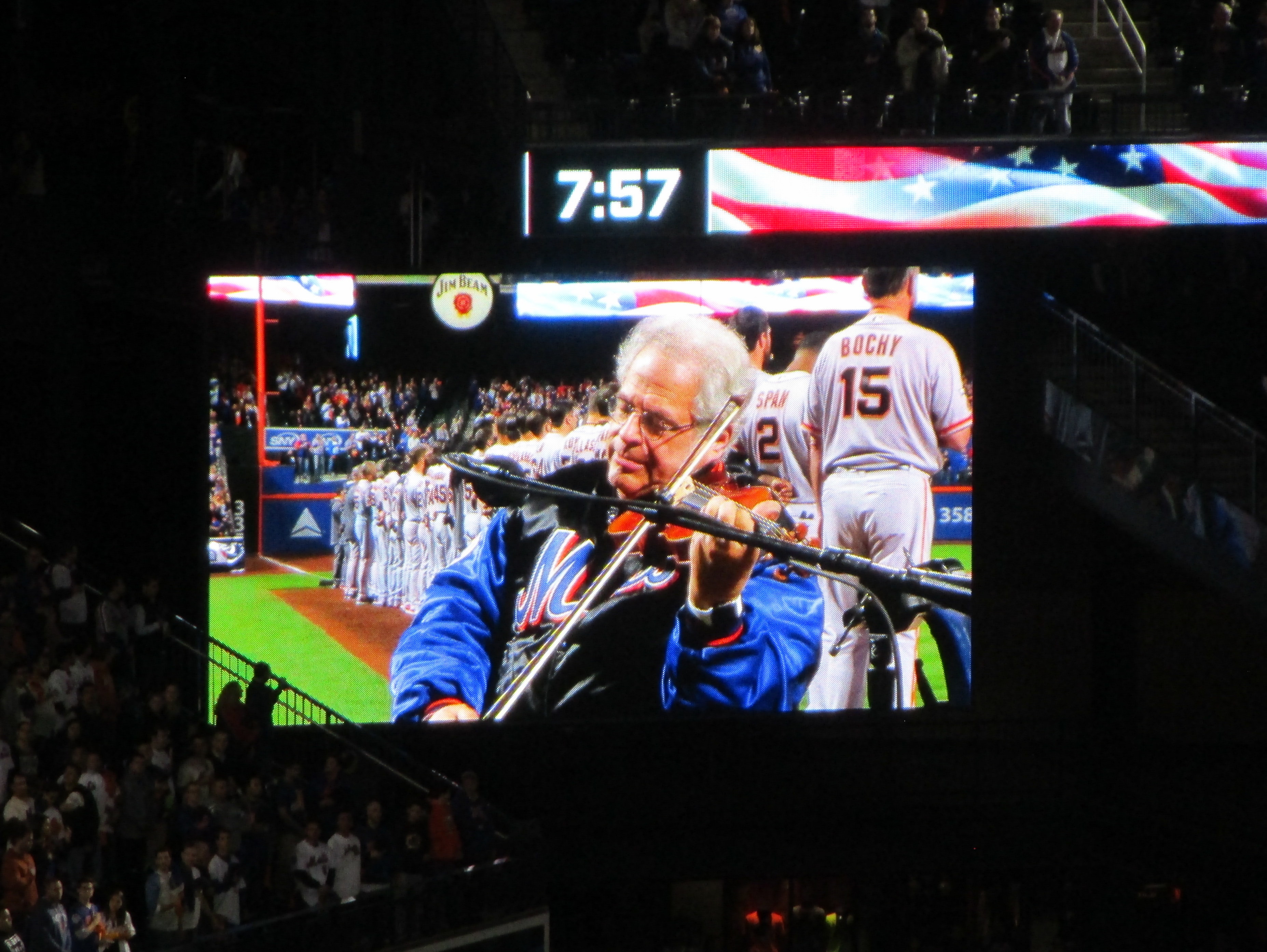In this detailed image, we see a large screen at a Major League Baseball game, suspected to be a San Francisco Giants game. The focal point is an older man with gray hair and wearing glasses, captured playing the violin, perhaps performing the national anthem. He's dressed in a distinct Mets jacket, colored blue and black with red accents. Positioned in front of or behind him, the team members are lined up along the baseline, visible from the back in their standard uniforms. The scene takes place at 7:57, as indicated by white numbers on the screen, which also displays an American flag. Behind the man, the stadium's stands are filled with spectators, and we can see sections of seated people. Additionally, there is a flag banner at the top of the screen, a television logo in the top corner, and a black microphone positioned in front of the violinist, adding to the ambiance of this patriotic and communal moment at the ballpark.